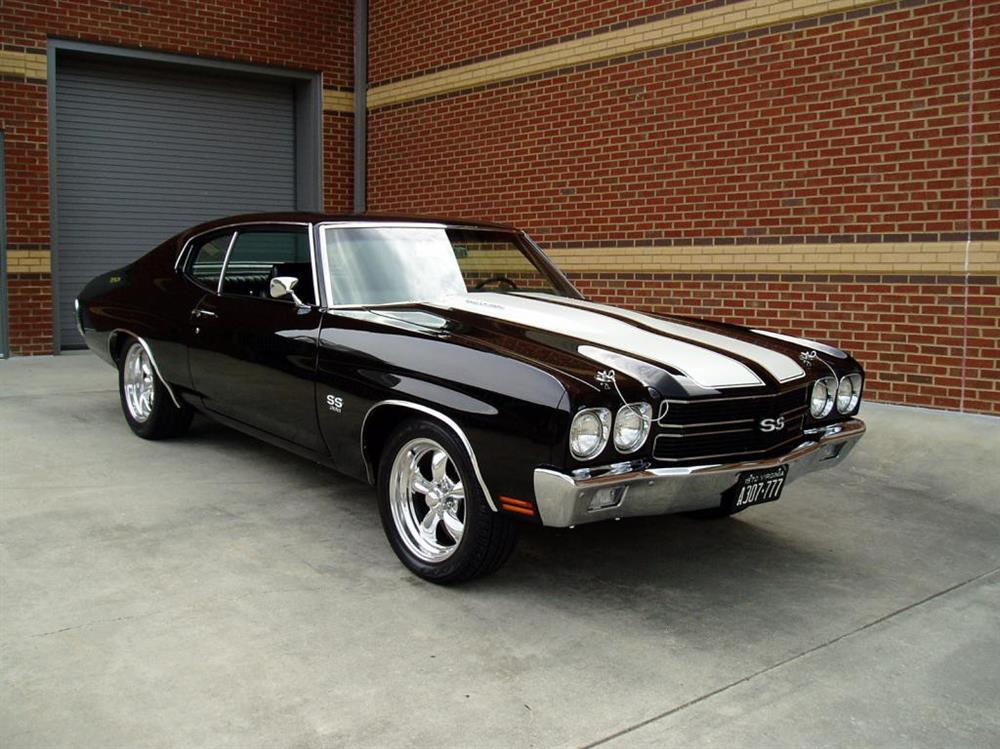The image features a striking, vintage muscle car, predominantly black with a white racing stripe running down the middle of the hood. At the forefront of the image, the car displays four prominent headlights and a chrome bumper, with an "SS" insignia centered on the grille. The design elements suggest it is a classic model, likely from the 1970s. The car, positioned on a gray concrete surface, faces right, revealing the shiny black passenger side along with silver hubcaps on black wheels. Red racing stripes adorn the front bumper, and another "SS" emblem is visible behind the front wheel on the side panel. The backdrop includes a red brick wall interspersed with yellow and beige bricks for trim, along with a gray garage door to the left.